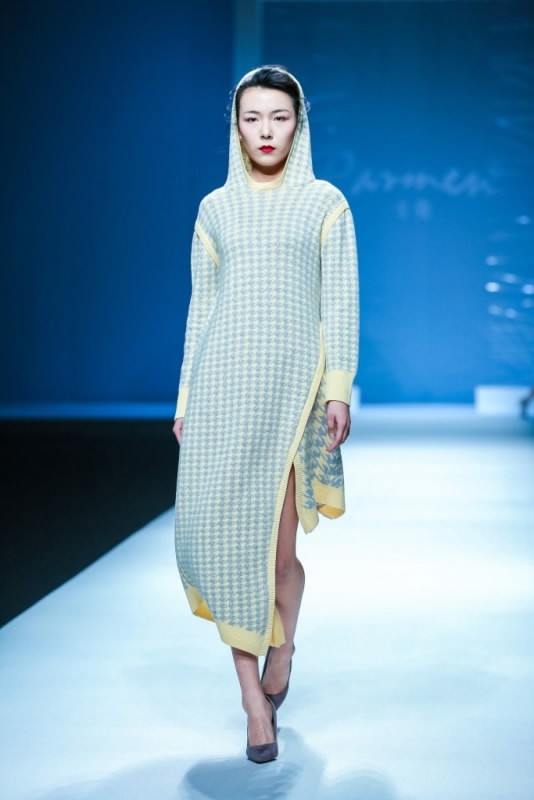This photograph captures an Asian female model confidently walking down a white runway during a fashion show. Behind her, a blue wall frames the scene, decorated with a light blue, unreadable word, possibly a designer's logo. The model, with black hair mostly hidden under her hood, sports a light blue and yellow houndstooth sweater dress that showcases intricate details. The dress features long sleeves, a hood, and a distinctive asymmetric hemline; it’s very long on the front and right side, reaching below her knees, while the left side is cut short above her knee. She accessorizes her look with striking red lipstick and dark gray high-heeled shoes. To the left of the runway is a dark gray floor, emphasizing the bright walkway. The model’s poised demeanor highlights the elegance of the ensemble, drawing viewers into the chic atmosphere of the show.